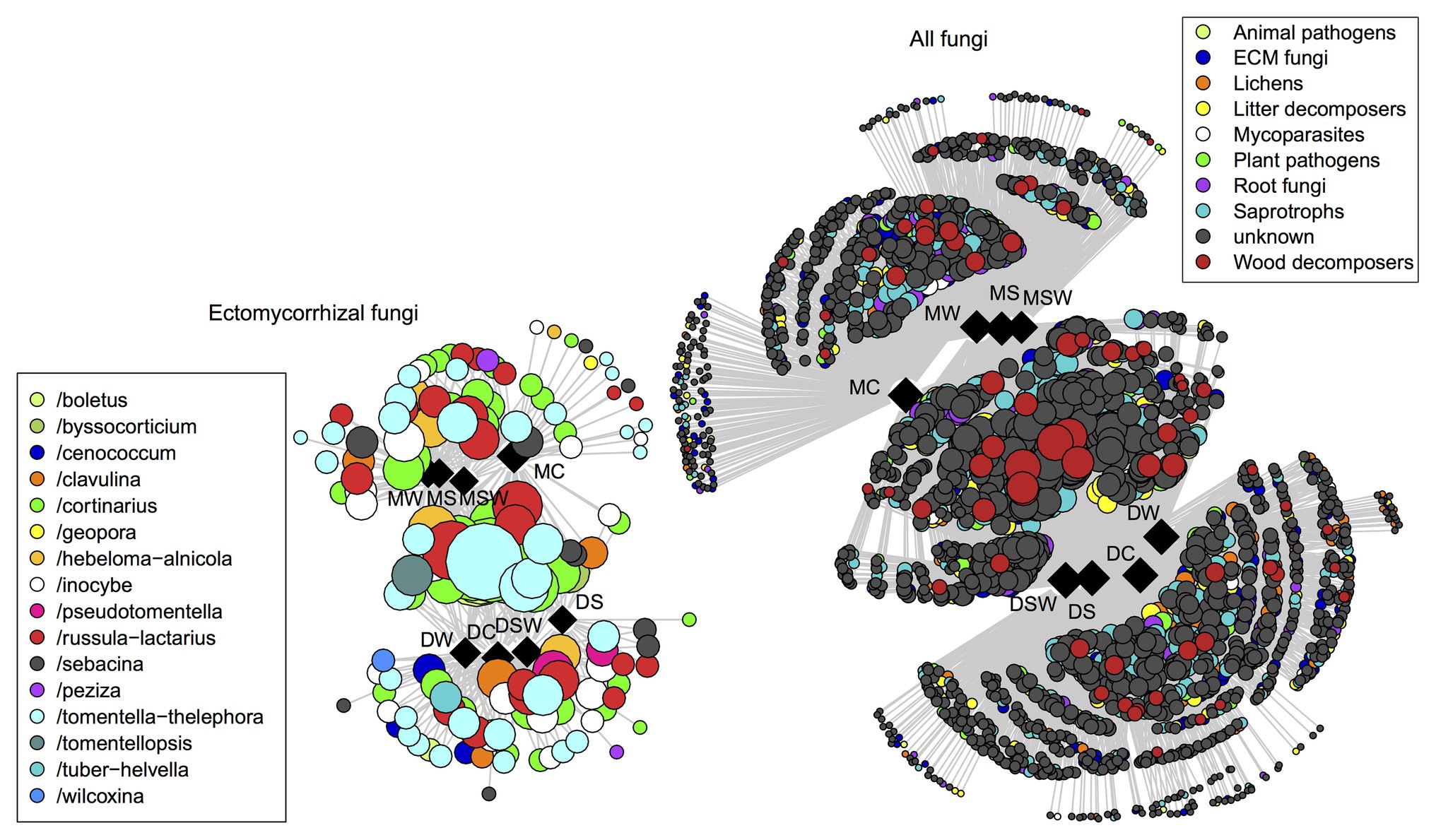The image depicts a detailed data visualization chart divided into two main segments, each adorned with circles of varying sizes and colors. On the left side, a cluster of brightly colored circles—light blue, green, yellow, light gray, white, red, and dark blue—represents different data points. Above these circles, the text "ectomycorrhizal fungi" is prominently displayed in black, with examples such as boletus, bisocordicium, and cynococum listed. Adjacent to this cluster is a rectangular key that explains the meaning behind each color.

On the right side, the image features another group of circles, predominantly gray, with some red, yellow, blue, and green. This section is labeled "all fungi," and includes associations like yellow for animal pathogens, black for ECM fungi, and orange for lichens. Similarly, a corresponding rectangular key on the right explains these color codes. Both segments feature black squares with initials like DW, DC, and DSW, which are likely explained by an external key not included in the image. The entire visualization is set against a white background, giving a clear view of the data presented.